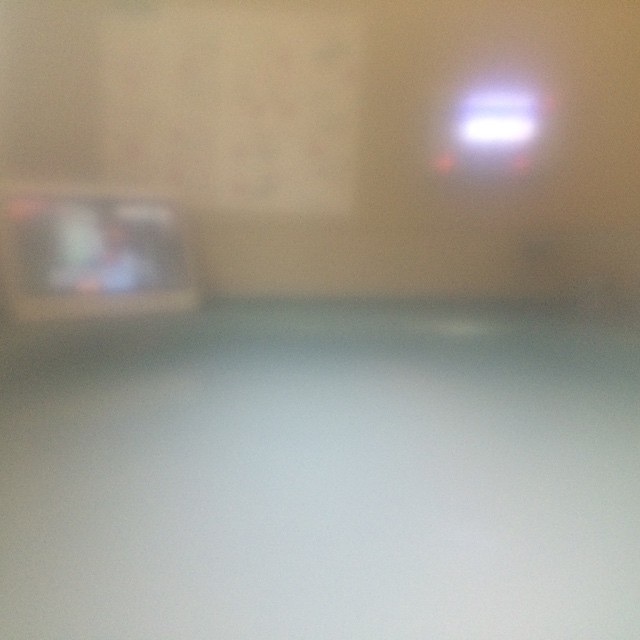A highly blurred photograph depicts what appears to be an operating or medical tech room. Despite the lack of clarity, a light blue bed or surface, possibly a patient bed, is visible in the foreground where the viewer seems to be positioned. To the left, a medical monitoring system is discernible, alongside another similar device in the background, resembling small television screens yet identified as medical equipment due to their appearance and arrangement. A large, indistinct chart or picture hangs on beige-colored walls, contributing to the room's clinical ambiance. The lighting is dim, primarily emanating from window blinds rather than overhead fixtures, casting shadows that obscure further details. The scene suggests a typical hospital environment with prevalent beige and light blue hues that evoke a sterile, medical atmosphere.